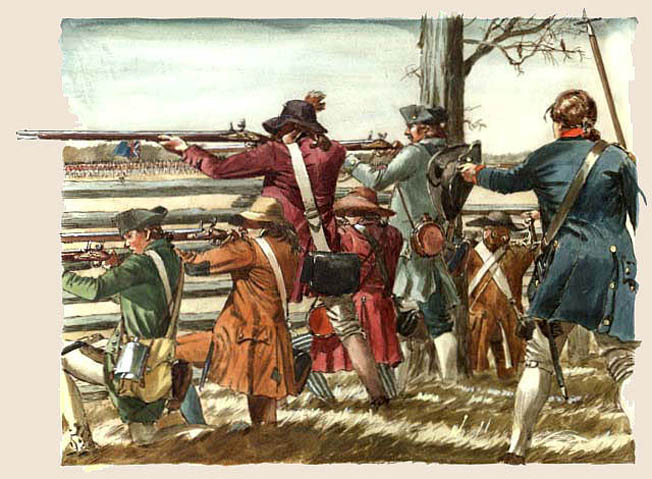The image portrays a detailed watercolor painting likely depicting a Revolutionary War scene. The painting, which appears to be on cloth or canvas with jagged edges, is mounted on a piece of backing paper, allowing the illustration to extend beyond the ripped edges. 

At the center of the composition, a group of seven soldiers, clad in various vibrant coats of navy blue, brown, burgundy, turquoise, and dark green, are positioned behind a wooden fence, armed with long muskets aimed towards the left. The soldiers, donning a mix of tricorn hats, large brimmed hats, and some with ponytails, appear to be preparing for a skirmish, evident from their crouched and kneeling stances.

On the right side of the painting stands a lone, leafless tree, adding to the stark, wintery atmosphere. Behind the line of soldiers is a commanding officer wearing a long blue coat, white leggings, and leather strap across his chest. He holds his hat aloft in his left hand while gripping a rifle in his right, with a sword at his side, seemingly directing the men.

In the vast distance, a phalanx of soldiers, distinguishable by their red shirts and white pants, represents the opposing British Army, marching towards the scene. Their figures are vaguely rendered with small dots of paint, emphasizing the distance.

The painting's border transitions into a light pink or off-white color, creating a soft frame that contrasts the vividness of the depicted wartime tableau.